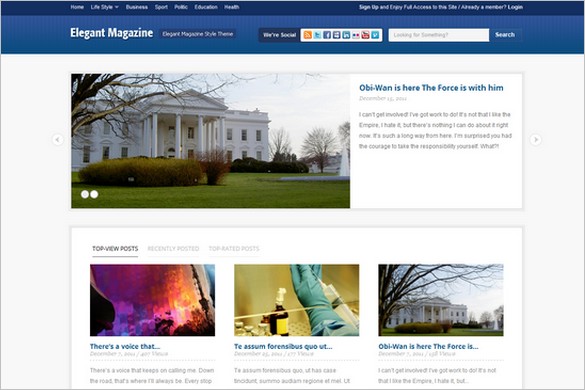This image is a screenshot of a webpage from the "Elegant Magazine" website. At the top left corner, there is a light blue bar featuring the title "Elegant Magazine" in white text. Above this bar is a darker blue navigation menu bar that spans across the width of the page. Below the light blue bar, in smaller white text, the phrase "Elegant Magazine Style Theme" is displayed, denoting the website's styling. To the right of this phrase, there is a reference to something social, followed by a series of social media icons. Additionally, there is a search bar positioned on the far right. Below these bars, the main content area is white, featuring prominently a photograph of a house. Accompanying the image, on the right side, there is a caption that reads, "Obi-Wan is here. The Force is with him."